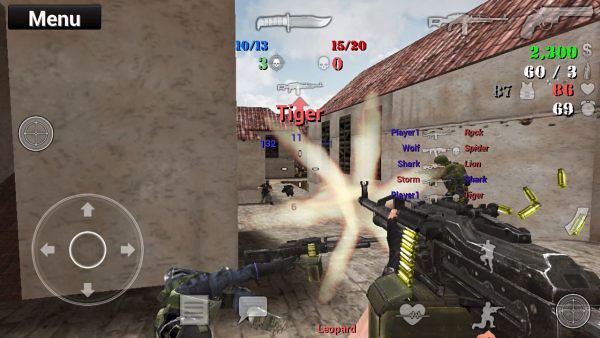This image is a detailed screenshot from a first-person shooter mobile game, which seems to evoke the graphical style of the early 2000s or late 90s. The player wields a large, belt-fed machine gun, complete with a massive drum and chain of bullets feeding into the weapon from the left side, as empty cartridge casings eject from the right. A vivid muzzle flash bursts from the barrel, illustrating the gun in mid-fire. The heads-up display (HUD) is rich with information: 

- In the bottom left corner, there's a control circle for character movement.
- The top left corner features a menu button labeled "menu" in white text on a black background.
- The bottom right prominently displays the player’s current weapon, a light machine gun, with its operational details vividly animated.

The background depicts a courtyard area with buildings, and the gun is aimed downrange towards three characters. Overhead, additional HUD elements show various weapon outlines, health, armor, and monetary values. Text includes numerical stats in blue and red lettering (e.g., "10/13" and "5/20") and the word "Tiger."